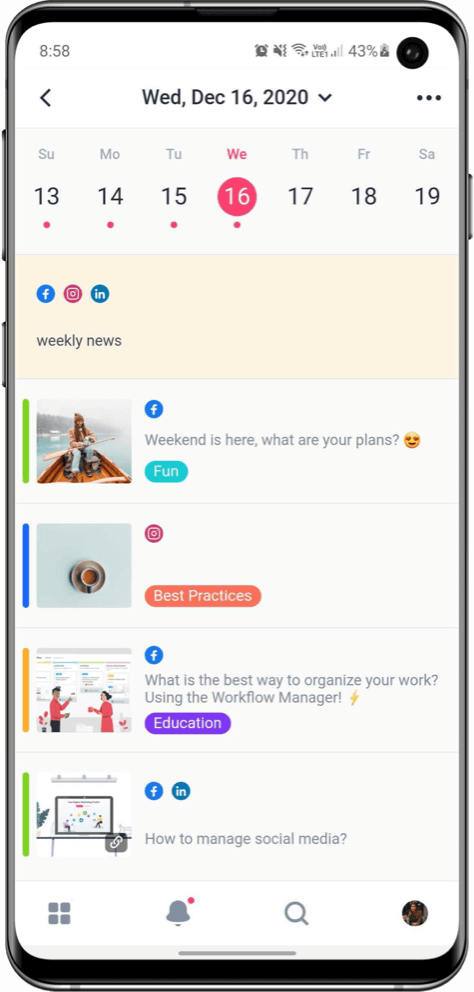Here is the cleaned-up and detailed caption:

This photo showcases a smartphone screen with a black border, thicker at the top and bottom. The center of the screen is white. In the top-left corner, the time reads 8:58. The top-right corner features a black circular icon, followed by a battery icon showing 43% charge. Next to it, the cellular signal indicates two out of four bars, labeled LTE. The Wi-Fi icon shows a full signal, alongside silent mode and alarm icons.

Below this, the screen displays a bar with a left-pointing greater-than sign, an ellipsis on the right, and the text "WED, December 16, 2020" in black, with a greater-than sign pointing downward. A gray border follows, listing the days of the week from Sunday to Saturday. Below this, the dates 13, 14, 15, and 16 are shown in black, except for Wednesday, which has a pink background, a white 16, and a pink dot underneath.

Below this day's navigation, there's a thin pink border containing icons for Facebook, Camera, and LinkedIn, beneath which is the text "Weekly News" in black. The remaining screen is white with four pictures aligned on the left and related information on the right. Each of the four pictures is bordered differently: the top picture has a green border, the second has dark blue and orange, the third has dark green, and the fourth at the bottom comprises four small squares forming a large square.

At the bottom of the screen, icons for notifications and search are visible, with the user’s profile picture in the bottom-right corner.